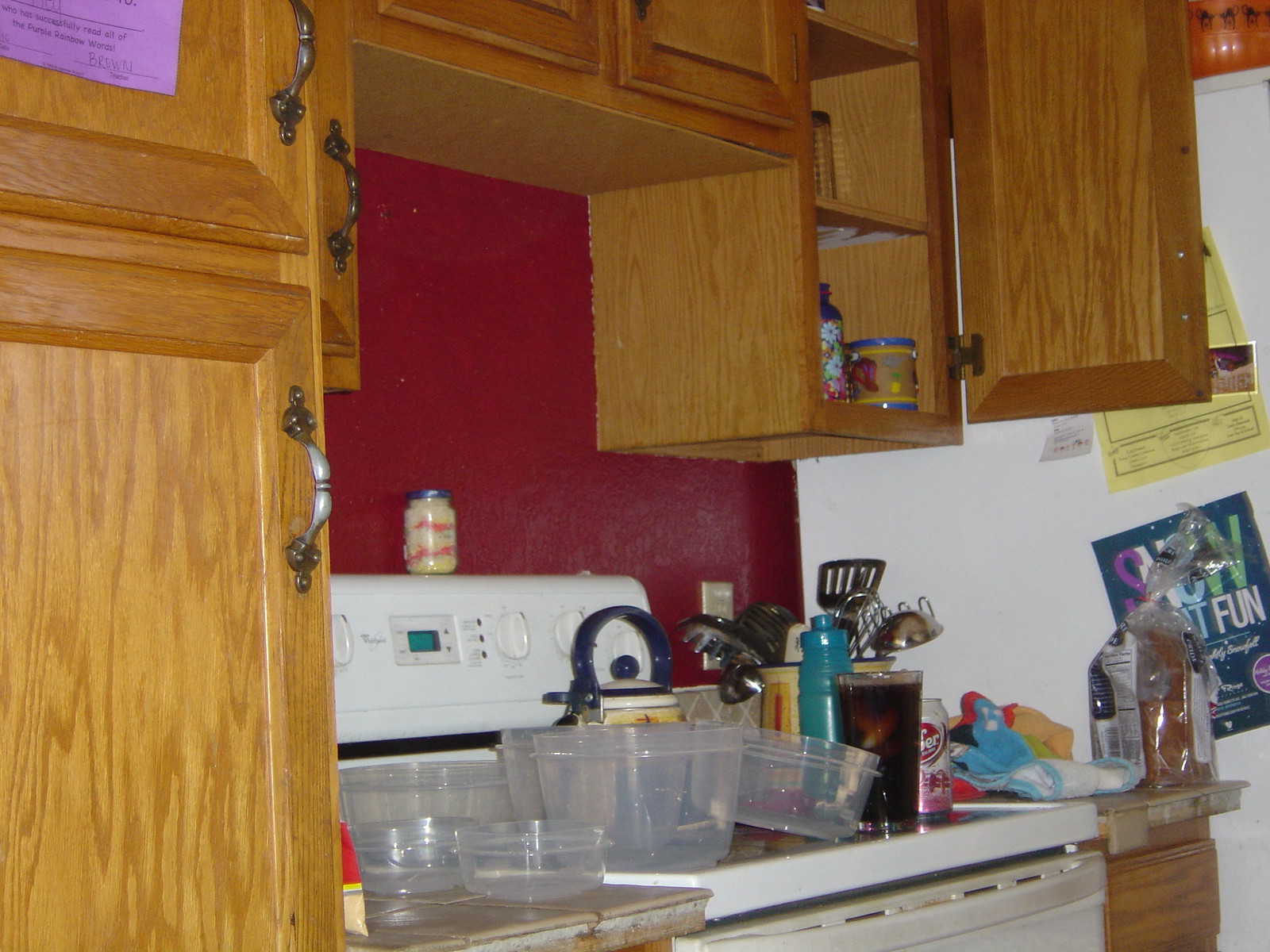A brightly lit kitchen snapshot focuses on the cabinetry framing a white range, extending to the adjacent side of a refrigerator. The oak cabinets, adorned with vertical pulls, feature a medium brown stain with a clear finish. The backsplash behind the stove is painted a glossy dark red, adding a pop of color to the scene. 

Atop the stove, a mason jar filled with layered contents sits near the back, surrounded by various items. A Dr. Pepper drink with ice cubes, identified by a nearby can, rests on the stovetop alongside a tea kettle. Several plastic containers are also precariously placed on the stove, along with a utensil caddy brimming with stainless steel kitchen tools, including a spatula, potato masher, ladle, and a pasta scoop.

On the counter to the stove's right, an upright loaf of bread in a bag and some potholders are visible. Above this narrow counter, an open cabinet displays its contents: a glass on the middle shelf, with several mugs on the bottom shelf. The side of the white refrigerator next to the range is adorned with papers held in place by magnets, completing this detailed glimpse into the kitchen's everyday setup.